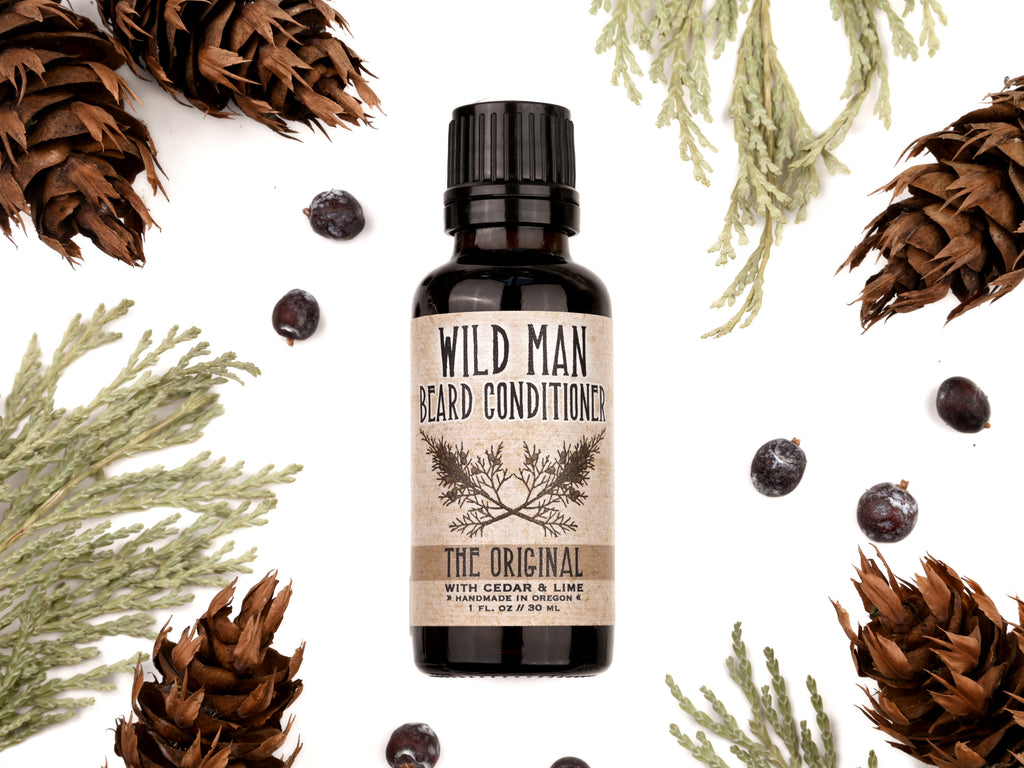This is a detailed advertisement for Wildman Beard Conditioner, specifically the original formula with cedar and lime, handmade in Oregon. The product is housed in a dark brown, glass bottle with a black cap, containing one fluid ounce (30 milliliters) of conditioner. The bottle features a light beige label adorned with artwork in shades of brown, gold, and beige. This artwork includes illustrated cedar branches and fir cones, contributing to a natural, rustic aesthetic.

The bottle is centrally positioned against a pale white background, creating a clean, minimalist look. Surrounding the bottle are various natural elements: in the top left corner, there are a couple of fir cones and cedar tips; moving towards the right, more cedar branches and additional fir cones are depicted. Juniper berries are scattered around, with another fir cone in the bottom right corner. Along the bottom edge, from right to left, are more cedar twigs, a couple of juniper berries, and another fir cone. Ascending from the bottom left corner is another cedar bough, complemented by a couple of juniper berries at the top. This arrangement frames the bottle and accentuates its natural ingredients, conveying a fresh and earthy vibe.